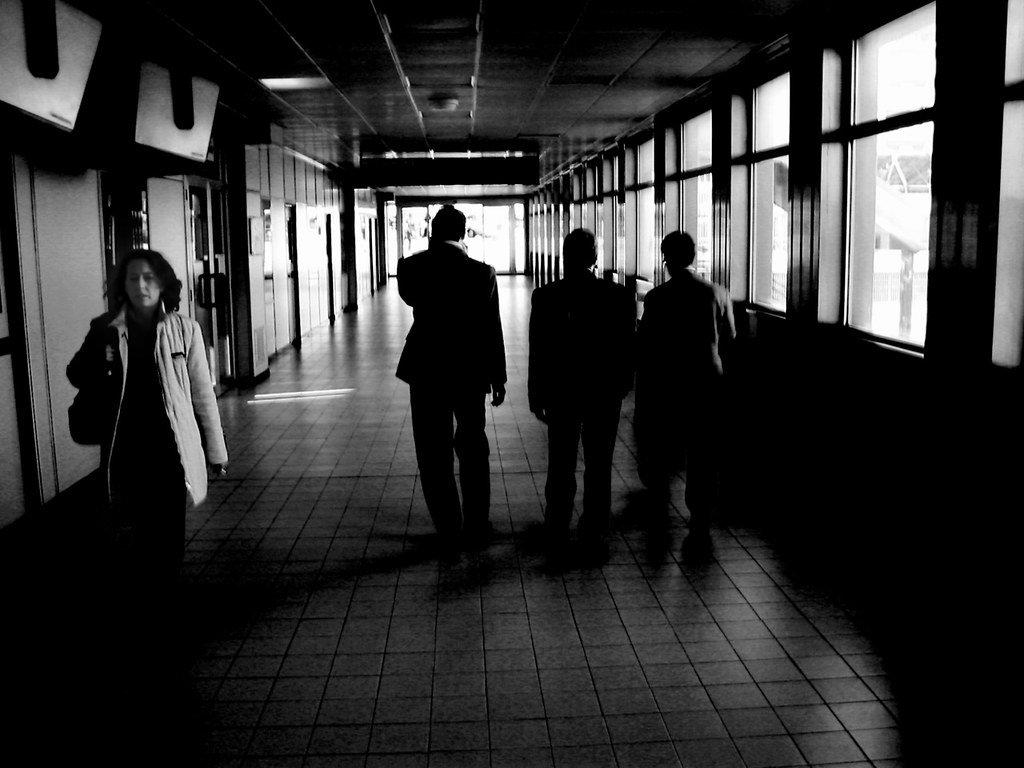This black and white image captures a dimly lit, long hallway, seemingly part of a public building or bus station. The floor is tiled and to the right, a row of half-height windows allows light to pour in, illuminating the otherwise shadow-filled corridor. The image features four individuals: three men walking away from the camera and a woman walking towards it. The men, all appearing to wear dark business suits, are of varying heights with the tallest on the left, the shortest on the right, and one in the center. One of the men appears to be on the phone. The woman, a Caucasian with dark or dark-blonde hair, strides purposefully towards the camera dressed in dark clothing with a light-colored coat, carrying a purse over her right shoulder. The hallway's left side is lined with doors, possibly leading to offices or other rooms. At the far end of the corridor, a door brightly lit from outside marks the exit, casting long shadows that enhance the image's stark contrasts. A single light fixture might be present above, though most of the illumination emanates from outside light coming through the windows.